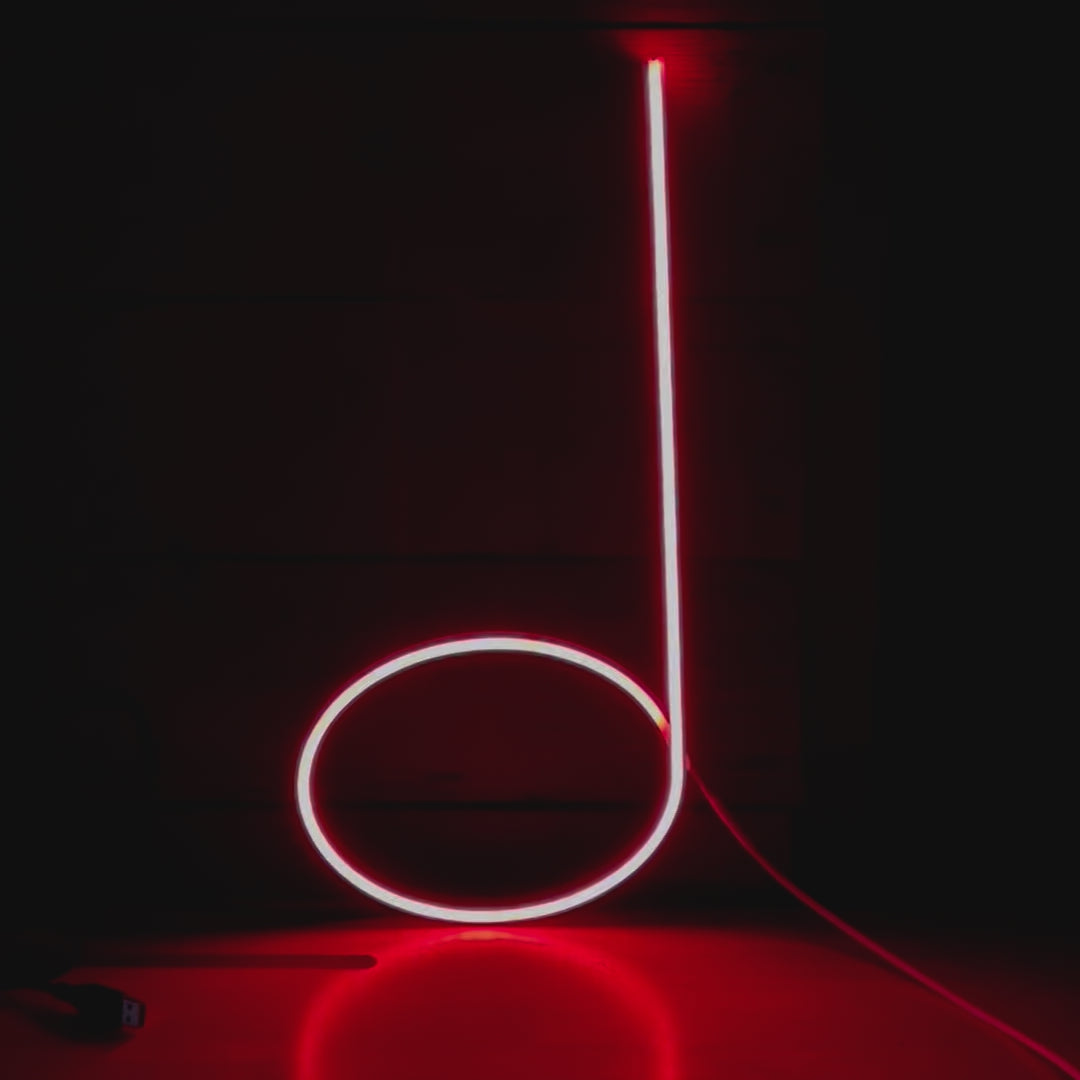In the dark room, a neon light strip emits a vibrant pinkish-reddish glow, creating a striking contrast against the black background. The flexible LED light is shaped like a lowercase 'd', with a horizontal oval forming the main body and a straight line extending upwards on the right side. This illumination is intense at the top, tapering off towards the bottom where the 'd' shape transitions into a darker tail. The light reflects faintly on the surface in front of it. A wire protrudes from where the curve of the 'd' meets its back, sloping off to the right and out of the frame, and suggesting it is plugged in and leaning against the wall. On the bottom left corner of the image, the edge of a USB plug is faintly visible, adding to the minimalistic composition.